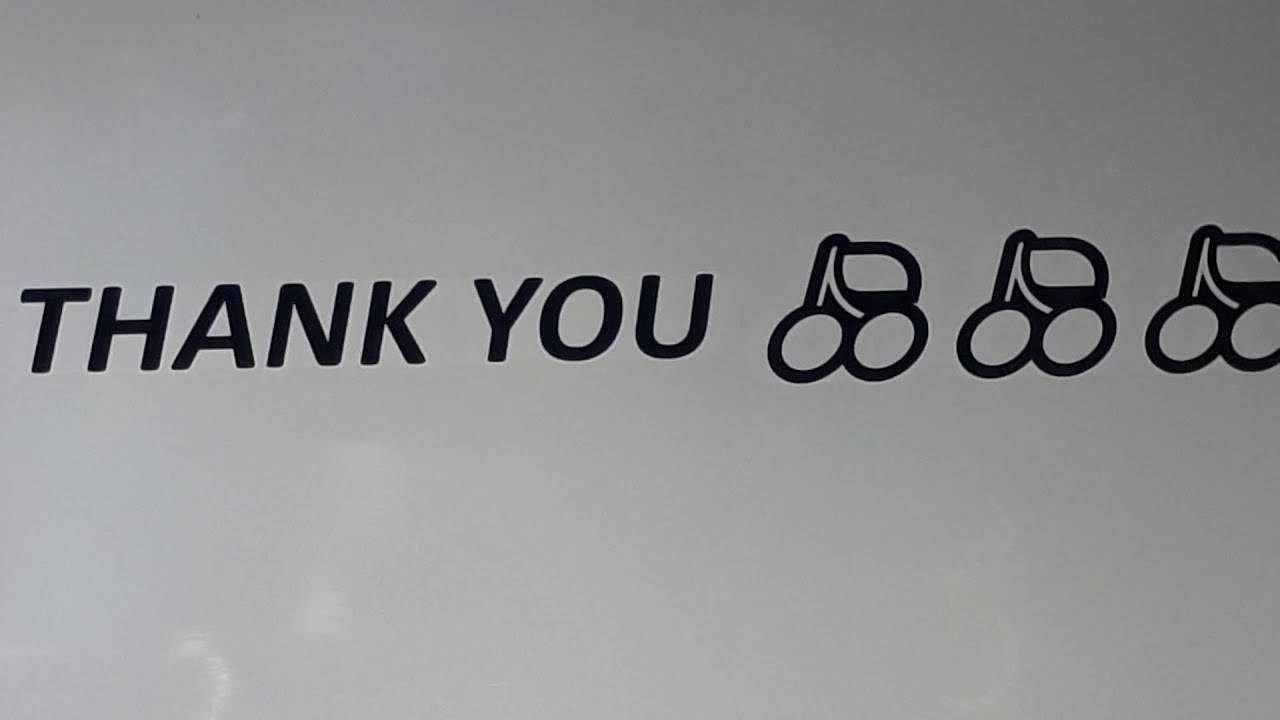In the partial view of the screenshot or design logo, there is a simple yet visually engaging composition. The main elements are set against a primarily white background that subtly transitions to gray, particularly more pronounced on the left side. Central to the image is the phrase "THANK YOU," written in bold, black, and slightly tilted text. Accompanying the text are three computer graphic images of cherries, each outlined in black. The cherries resemble stylized icons from classic video games like Pac-Man, consisting of a central twig running vertically with a small rectangular shape on one side acting as a leaf. The main twig extends downward to form a Y-shape with two circles representing cherries at the ends of the branches. These cherry graphics are evenly spaced to the right of the text, although the third cherry on the far right is slightly cut off. The screenshot measures about nine inches wide by five inches tall and is of relatively poor quality, with some reflective areas affecting the clarity. The image is devoid of any other objects, people, or borders, adding to its minimalist and focused design.